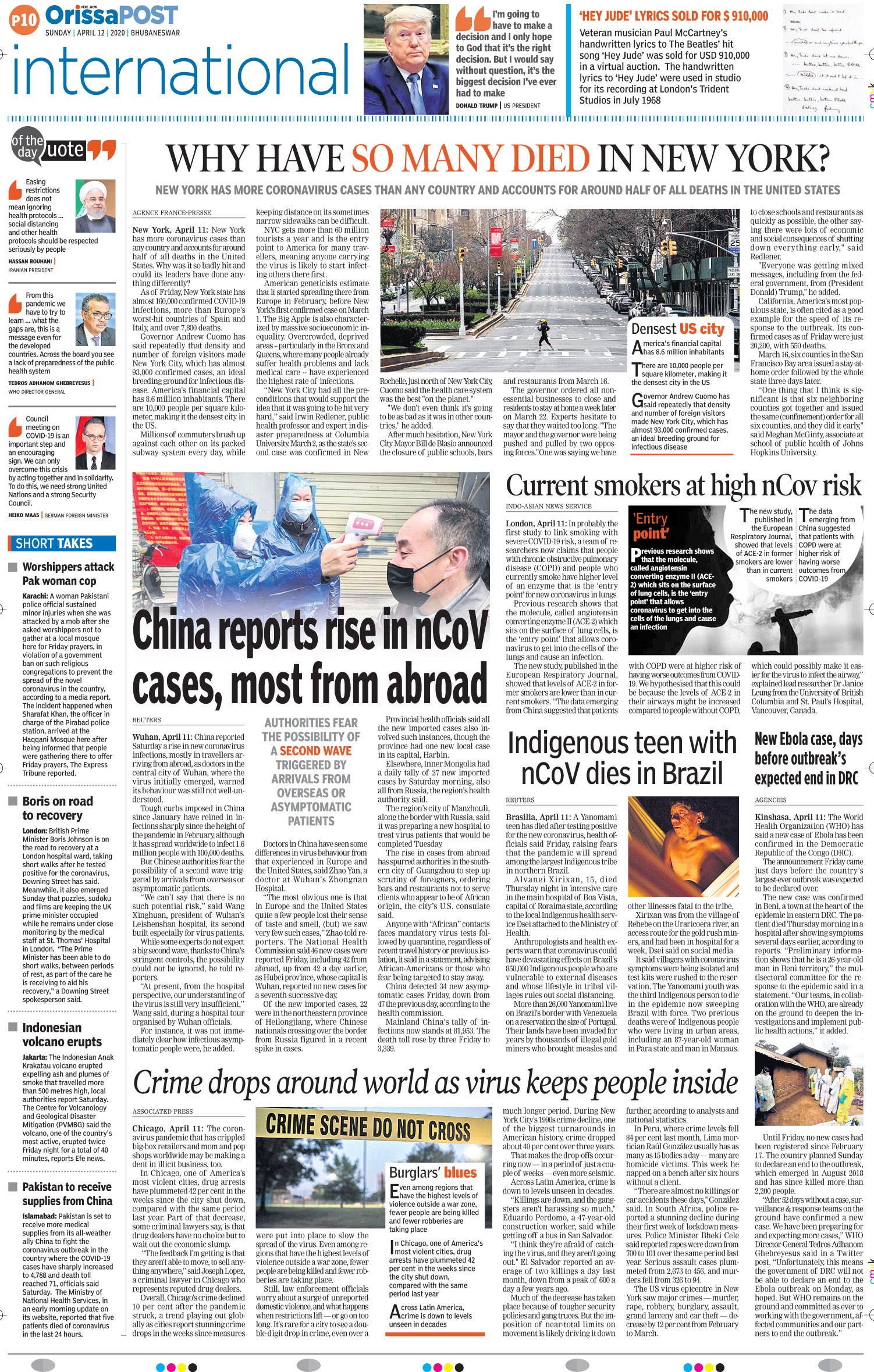**Arisa Post – Sunday, April 12th, 2020 (International Section)**

![Screenshot of a Digital Newspaper Outline]

In the top-left corner, there is an orange circle with the text "P10" in white, alongside the publication name "Arisa Post" in blue. The date "Sunday, April 12th, 2020" is also visible.

**Main Headline: Why Have So Many Died in New York?**

- **Detail**: New York has more coronavirus cases than any country and accounts for around half of all deaths in the United States. 
- **Visual**: Image of a person running across an empty New York street.

**Secondary Highlights:**

1. **Hey Jude Lyrics Sold for $910,000**
   - **Detail**: Not much body text is readable.
   - **Visual**: Blue separator line and orange text for the heading.

2. **China Reports a Rise in NCOV Cases**
   - **Detail**: Most of the new cases are from abroad.
   - **Visual**: Images of people in protective suits with gun thermometers, all wearing masks.

3. **Current Smokers at High NCOV Risk**
   - **Visual**: Black and white image of a person smoking.

4. **Indigenous Teen with NCOV Dies in Brazil**
   - **Visual**: An unspecified image related to the story.

5. **Crime Drops Around the World**
   - **Detail**: The virus keeps people inside.
   - **Visual**: Image of a crime scene with "Do Not Cross" tape.

**Left Sidebar:**

1. **Quote of the Day**
   - **Visual**: Images of three different people with their respective quotes, although the text is not clear.

2. **Short Takes**
   - **Detail**: Additional smaller stories with unreadable text.
   - **Visual**: Includes various images.

**Footer:**

- **Printing Marks**: Cyan, Magenta, Yellow, and Black seen at the bottom, indicating this is likely a printing proof.

**General Notes**: The page layout reflects a typical newspaper format with multiple headlines, images, and separator lines, although much of the text is not readable. The visual elements suggest a comprehensive coverage of international news, particularly focused on the global impact of COVID-19.